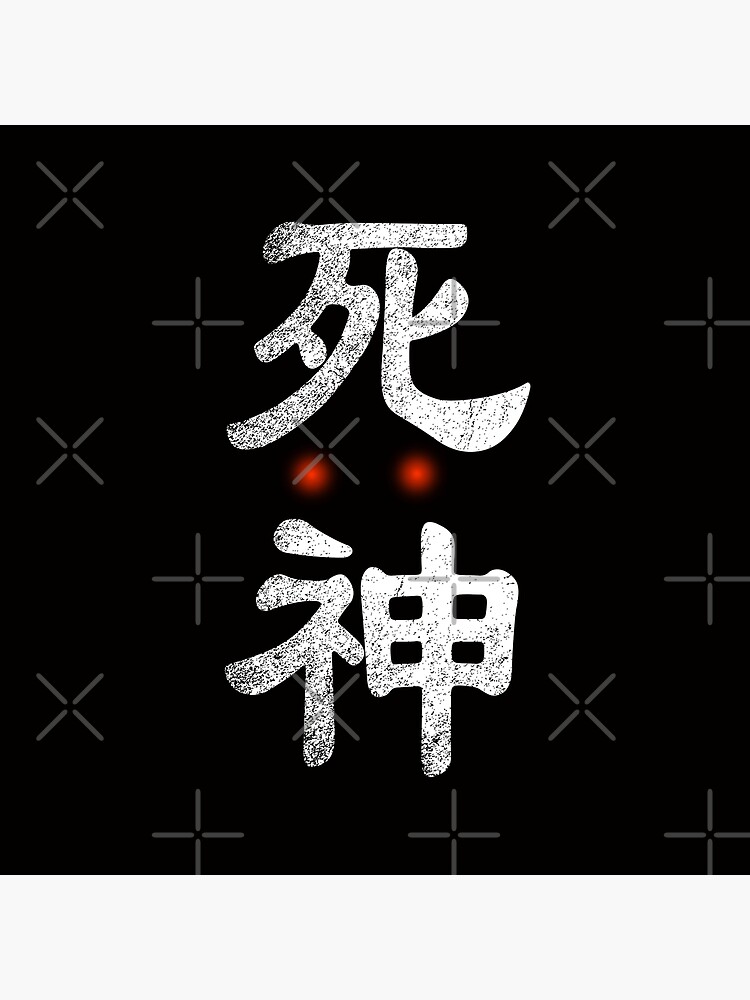The image features a black background with a soft, intricate pattern of silver X's and plus signs scattered throughout. Central to the image are two Chinese or Japanese characters, rendered in a sparkling, whitish-silver texture. One character is positioned at the top and the other at the bottom. Between these characters, two small, glowing red dots with blurry edges are situated, resembling eyes. The entire composition exudes a mystical and ethereal quality, enhanced by the vertical white lines embellishing the top and bottom of the image.